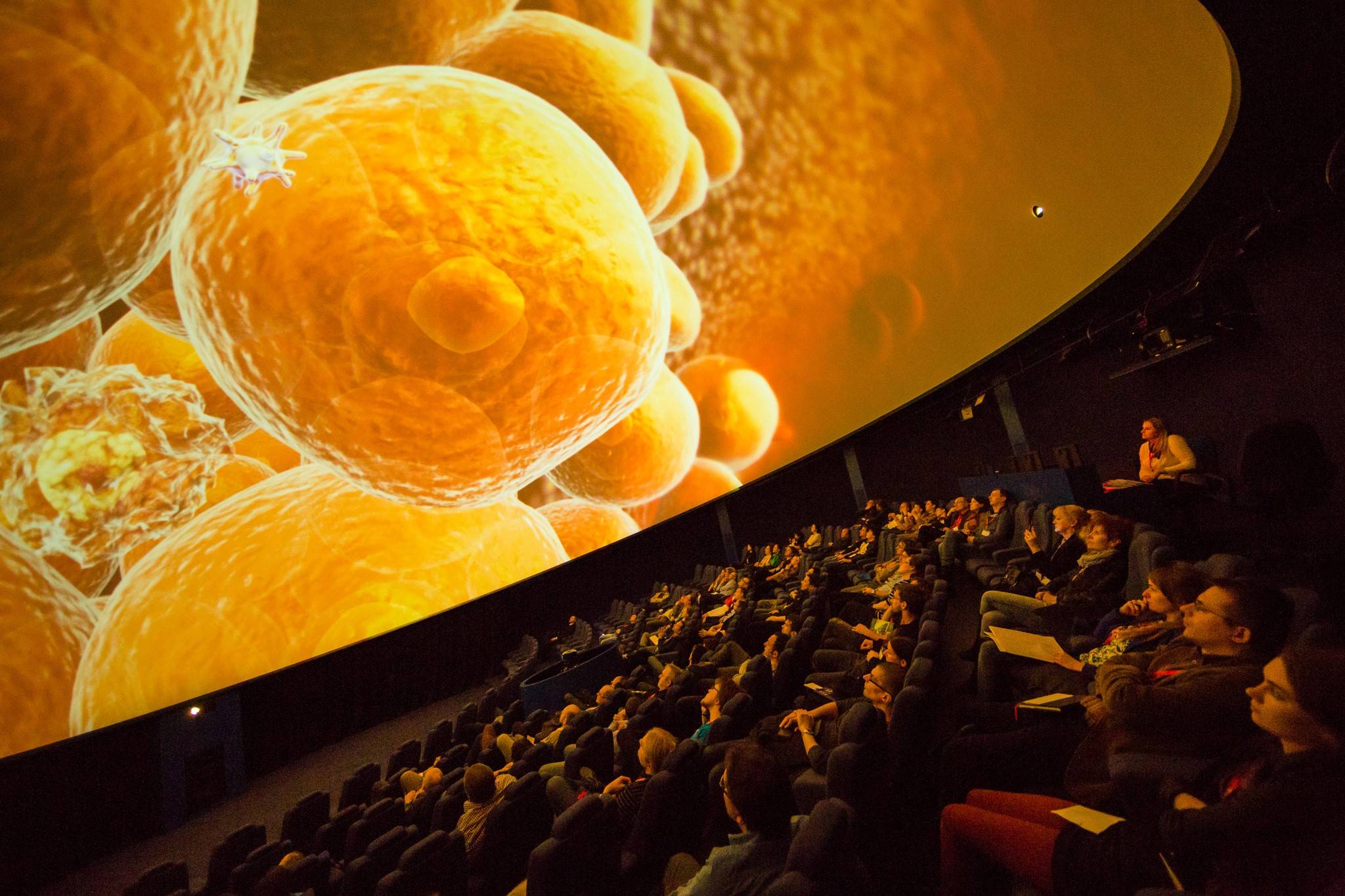The image depicts a large, curved auditorium with a domed ceiling, featuring a massive projection screen showing an intricate display of orange and yellow cell-like or molecular structures. The audience, consisting of over 50 people, is seated in a curved arrangement beneath the dome, intently observing the vivid projection. Small white lights accentuate the edges of the room, while a person positioned above the seating area appears to be managing the projection. The immersive, IMAX-style setup creates a striking visual experience for the attendees.